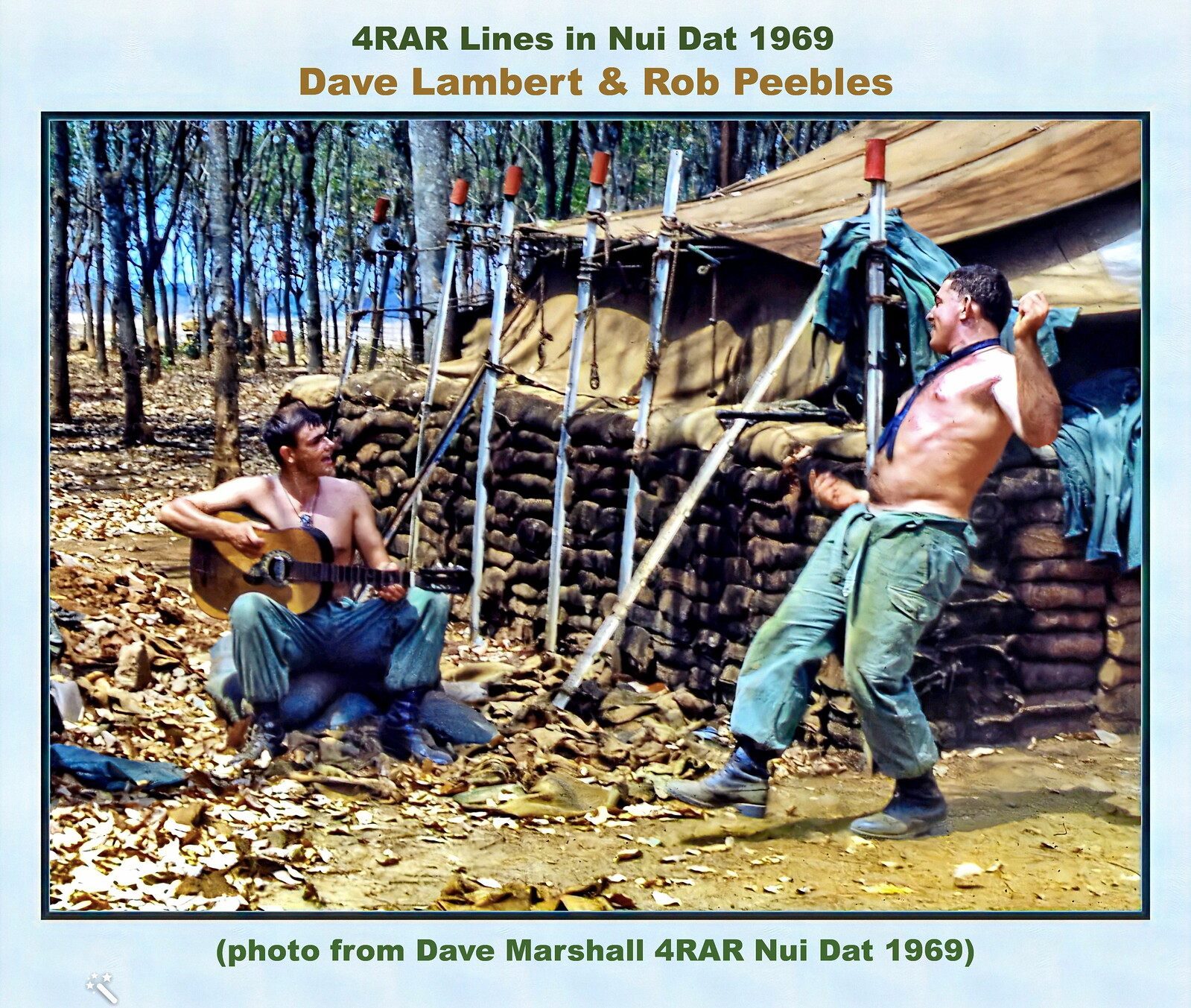In this detailed photograph, reminiscent of a postcard, captured in 1969 during the Vietnam War, two shirtless men, identified as Dave Lambert and Rob Peebles, are the focal point. They are surrounded by a rustic, woodland setting with a variety of slender trees in the background. The man on the left sits on the ground playing a brown guitar, while the other man stands to the right, seemingly dancing or leaning back. Both are wearing blue jeans. The setting appears to be an outdoor area with dirt and leaves covering the ground. Behind them is a large makeshift tent or wooden structure, possibly an army bunker, and a barrier constructed from logs. The image is framed with a blue border that includes text stating, "four RAR lines, Nouey Dot, 1969," and additional parenthetical details noting, "photo from Dave Marshall, four RAR, Nouey Dot, 1969." The overall scene captures a moment of camaraderie and respite amidst the war-torn setting.